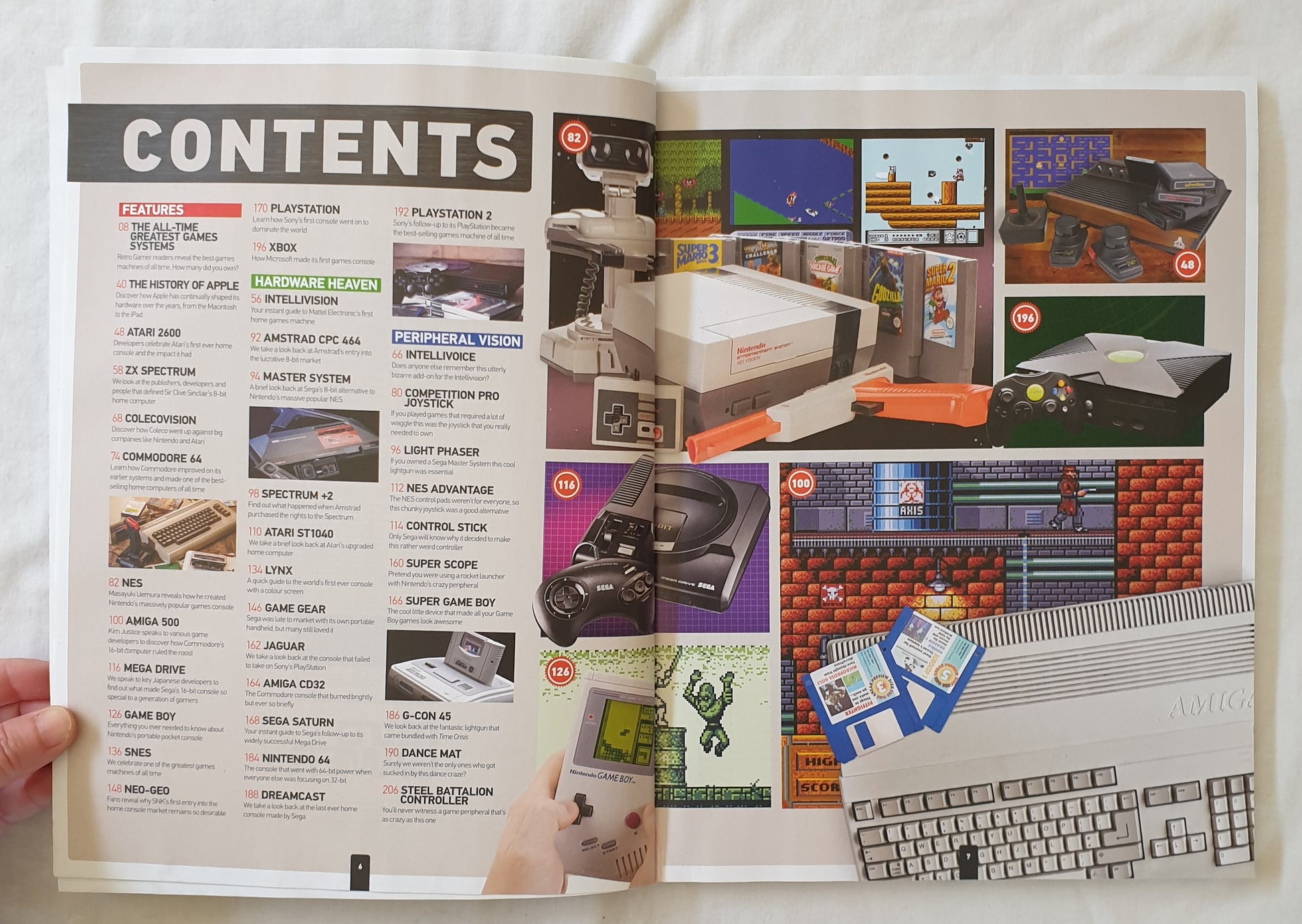This image is a photograph taken from the point of view of a reader looking down at an open magazine, specifically at its Table of Contents spread. The magazine, clearly focused on the history and evolution of gaming technology, is resting on a white bed sheet. A hand is seen holding the page open. The left page has a black bar at the top with "CONTENTS" written in a white, sans-serif, all-caps font. Below it, the sections are organized with colored bars—red for "FEATURES," green for "HARDWARE HEAVEN," and blue for "PERIPHERAL VISION," each listing various gaming consoles and peripherals such as the NES, Atari, ZX Spectrum, Commodore 64, Mega Drive, Game Boy, PlayStation, Xbox, Intellivision, Amstrad CPC 464, Game Gear, Sega Saturn, Nintendo 64, Dreamcast, and more. The right page features a series of numbered images corresponding to articles within the magazine, depicting iconic gaming systems and accessories like the NES, an original Xbox, a Game Boy, a Sega Genesis, an Atari system, a Virtual Boy, an Amiga, and a collection of floppy disks. These visuals, overlaid with red circles containing white numbers, guide the reader to specific contents inside the magazine. The overall setting suggests a casual yet informative deep dive into the historical facets of gaming.